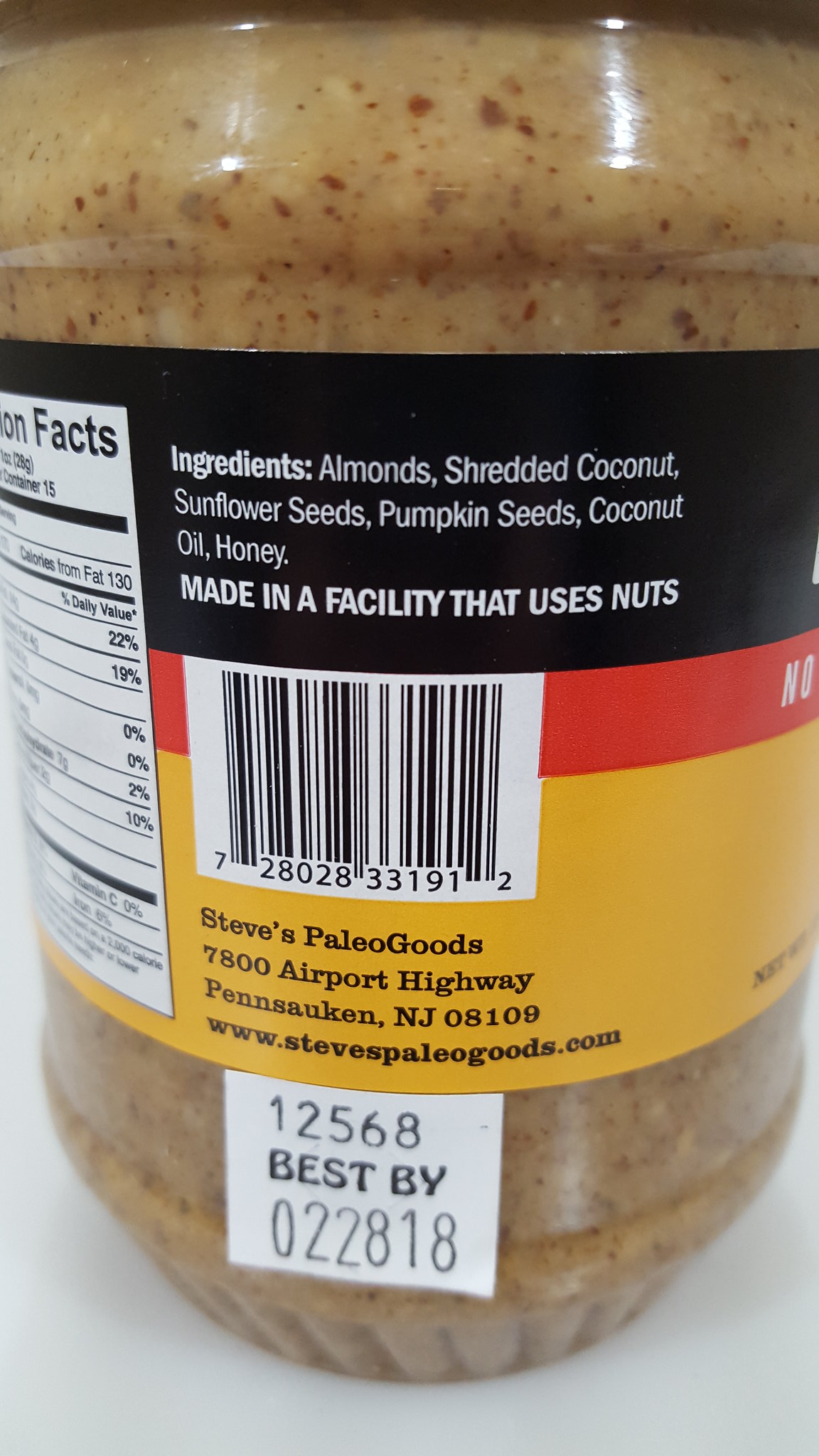This image showcases a package of canned food from Steve's PaleoGoods. The front label prominently lists the ingredients, which include almonds, shredded coconut, sunflower seeds, pumpkin seeds, coconut oil, and honey. An additional note indicates that the product is made in a facility that also processes nuts. The packaging includes a barcode and specifies the manufacturer's address: Steve's Paleo Goods, 7600 Airport Highway, Pennsauken, New Jersey 08108-1109. The company's website, www.stevespaleogoods.com, is also displayed twice for customer reference.